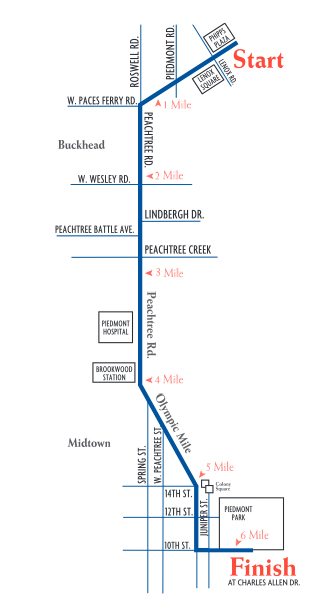This detailed map outlines a 6-mile route on a white background, marked by a prominent thick blue line indicating the main pathway. It starts at Phipps Plaza at the intersection of Lenox Road and Peachtree Road, highlighted in red text. All streets are labeled in small black text, with important intersections and mile markers noted by red arrows and labels. The route passes through key points such as Lenox Square, Piedmont Road, Roswell Road, and continues through major landmarks including W. Paces Ferry Road, Buckhead, W. Wesley Road, Lindbergh Drive, and Peachtree Battle. Each mile is clearly marked from 1 to 6 miles, spaced evenly along the route. Notable areas along the way include Peachtree Creek, Piedmont Hospital, Brookwood Station, Olympic Mile, W. Peachtree Street, Midtown, 14th Street, 10th Street, and Piedmont Park. The map ends at Charles Allen Drive, with a red text label indicating "Finish." This minimalistic map emphasizes the significant roads and locations, likely used for a public transportation route or a marathon.